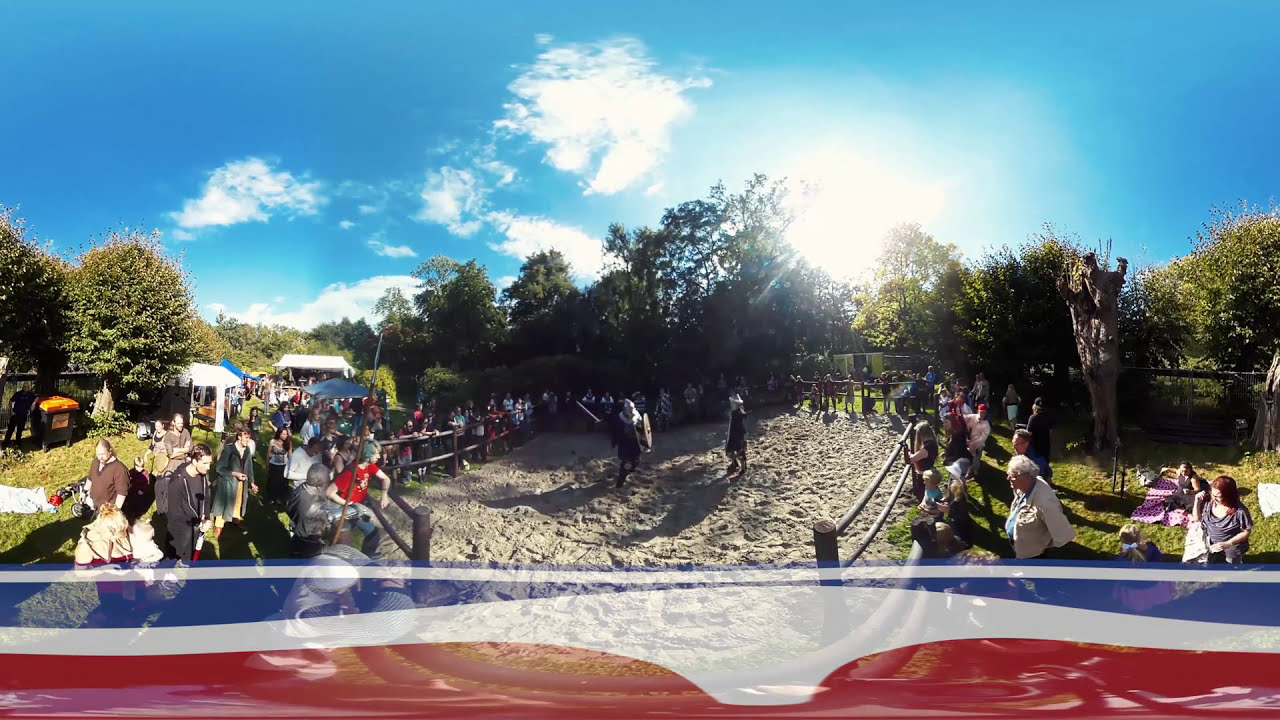The image captures a lively scene at what appears to be a Renaissance festival held in a rural, outdoor setting. The clear blue sky, sprinkled with sections of clouds and illuminated by the sun peeking through bushes and trees in the middle right portion, forms a picturesque backdrop. Central to the image is a large, well-trodden sandpit or corral, its light tan or beige surface surrounded by wooden fences. Within this arena, two individuals dressed as medieval knights appear to be engaged in a duel, complete with silver helmets and swords, though they seem to be in a momentary standstill.

The surrounding environment features a mix of forested areas and fields, suggesting a countryside locale. On either side of the corral, a diverse crowd gathers, with a denser assembly on the left compared to the right, all intently focused on the scene within the pit. The audience’s attire and the festive atmosphere hint at the event being a significant occasion for the town, drawing considerable interest. Adding a touch of national pride and further emphasizing the festival atmosphere is a translucent red, white, and blue banner draped along the bottom of the image. Also visible are some tents, possibly vendor stalls or makeshift shelters, enhancing the historical ambiance. The overall scene combines the nostalgic charm of both Old Western and medieval reenactions, brought together under a bright, tranquil sky.